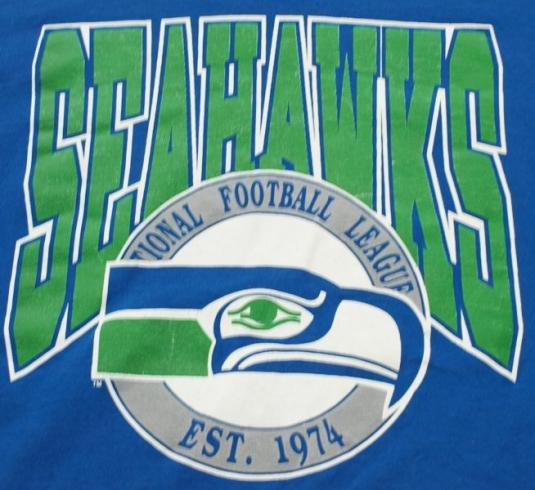This image is a photograph of a blue piece of clothing, likely a t-shirt or blanket, showcasing a Seattle Seahawks design. Dominating the upper portion of the image, bold green block letters outlined in blue and white spell out "Seahawks." Partially overlaying this text is a circular logo, featuring a gray ring with white in the middle. The logo displays a blue and green Seahawk facing to the right, with a green eye and a blue beak. Encircling the bird, the gray ring bears the text "National Football League" partially obscured by the logo, and "EST 1974" at the bottom, marking the establishment year of the franchise. The colors and design elements clearly reflect the iconic Seattle Seahawks branding.